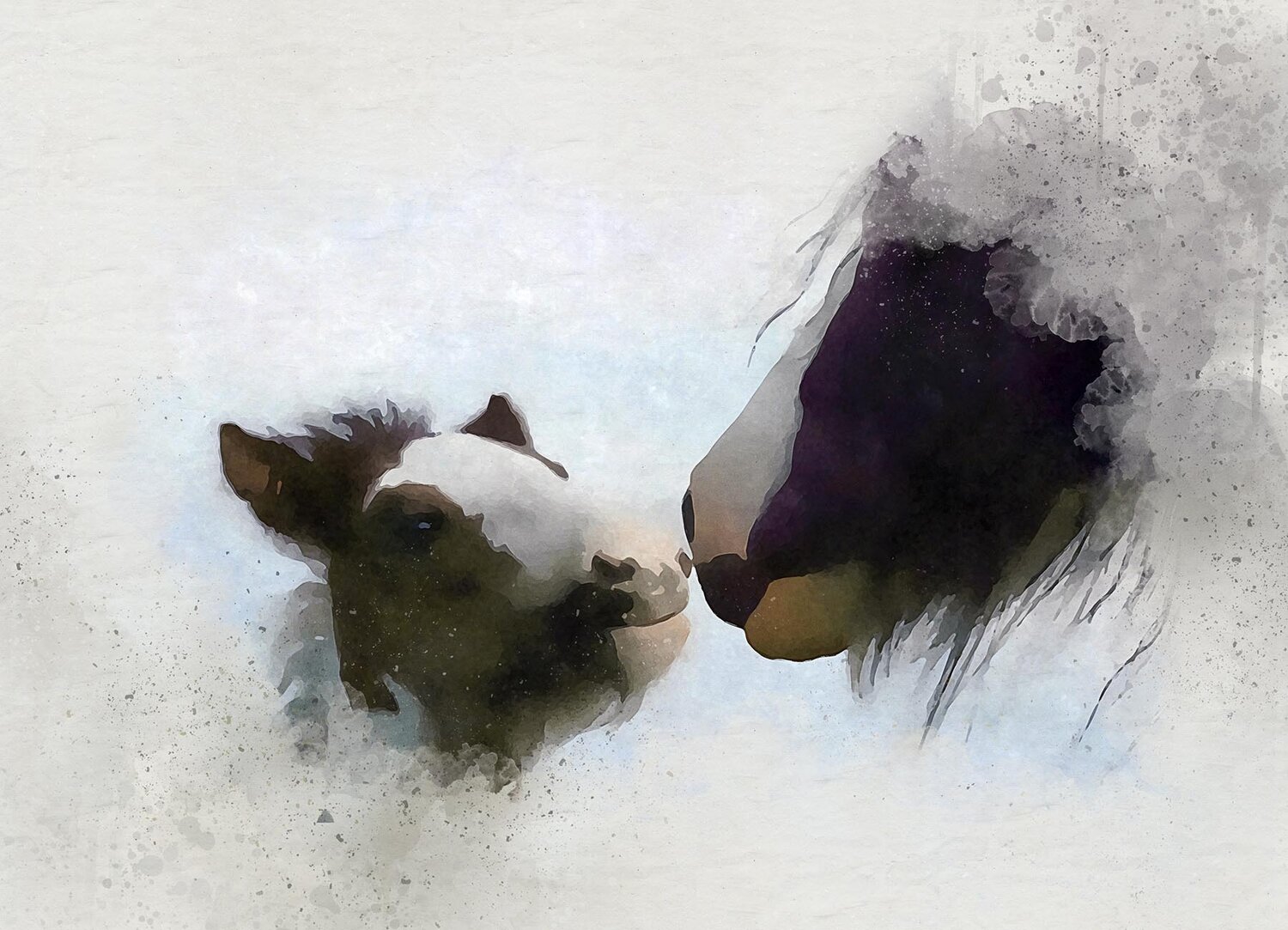This is a watercolor painting depicting a touching scene between a horse and a young cow, presumably a mother and her colt or calf. The composition focuses solely on their heads, set against a pale, off-white background with gray flecks that resemble snow. The adult horse, positioned on the right side, has a reddish-brown or purplish-toned head with long, shaggy hair, white markings on its jaw and nose, and is seen in profile. The young cow, or calf, situated to the left, has a predominantly brown head with a distinct white face and additional brown markings on its ears and cheeks. The background behind them is mostly white, with some hints of blue, emphasizing the connection between the two animals as their noses nearly touch. The painting's abstract style and sparse background draw attention to the intimate bond conveyed through their close interaction.